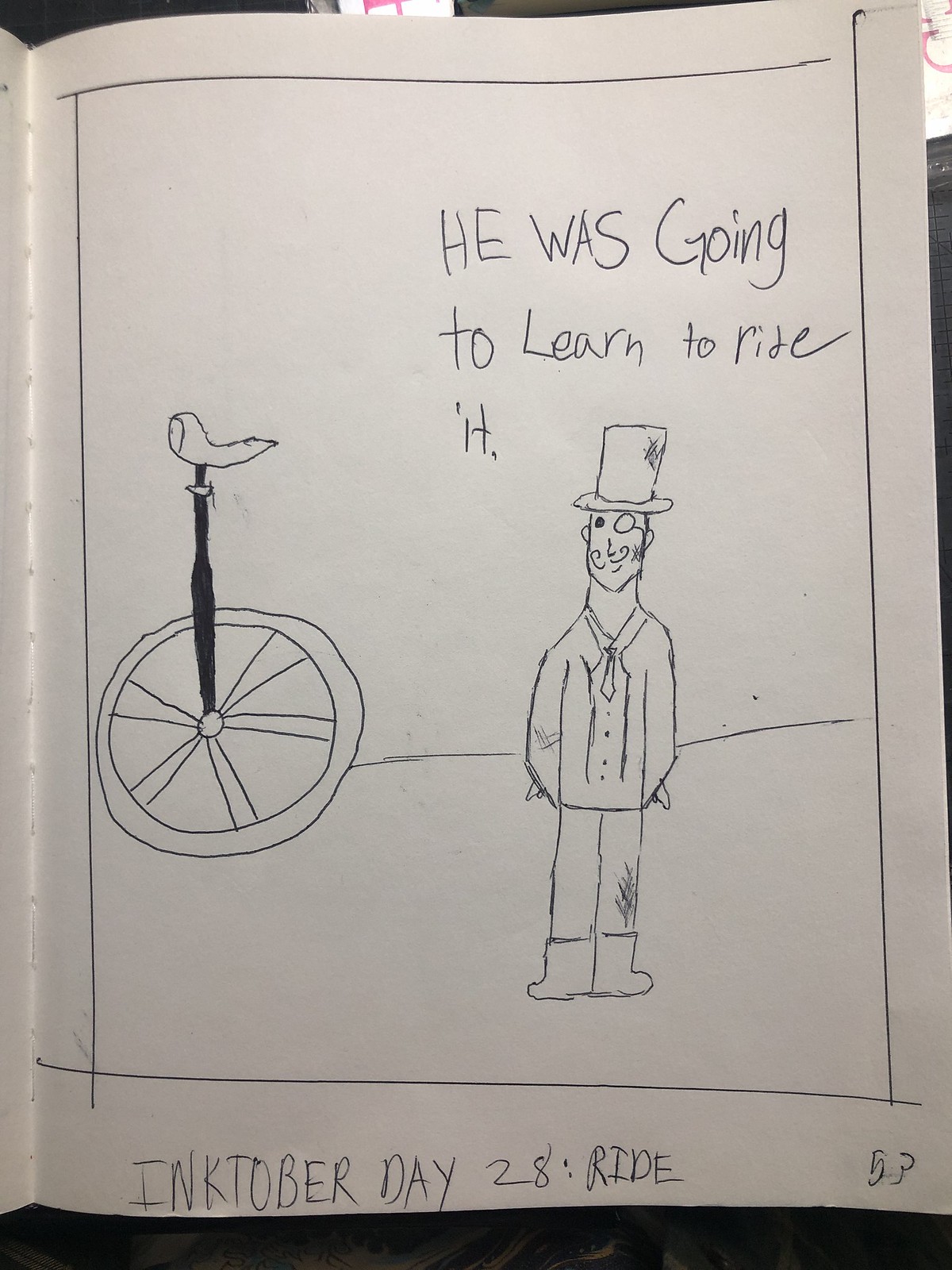On a white background, this detailed illustration is drawn entirely in black ink on a white paper. The bottom of the illustration reads "Inktober, Day 28: Call and Ride" in bold capital letters. To the right of this text, the number 53 is prominently displayed. 

In the middle left section of the image, a meticulously drawn unicycle features a seat and a wheel with detailed spokes. To the right of the unicycle, a distinguished man is depicted with a mustache, monocle, top hat, and tie, standing with his hands in his pockets and wearing formal shoes. 

At the very top of the image is a text box with the phrase, "he was going to learn to ride it," indicating the gentleman's intention. A horizontal line stretches across the scene, forming a horizon and adding depth to the composition.